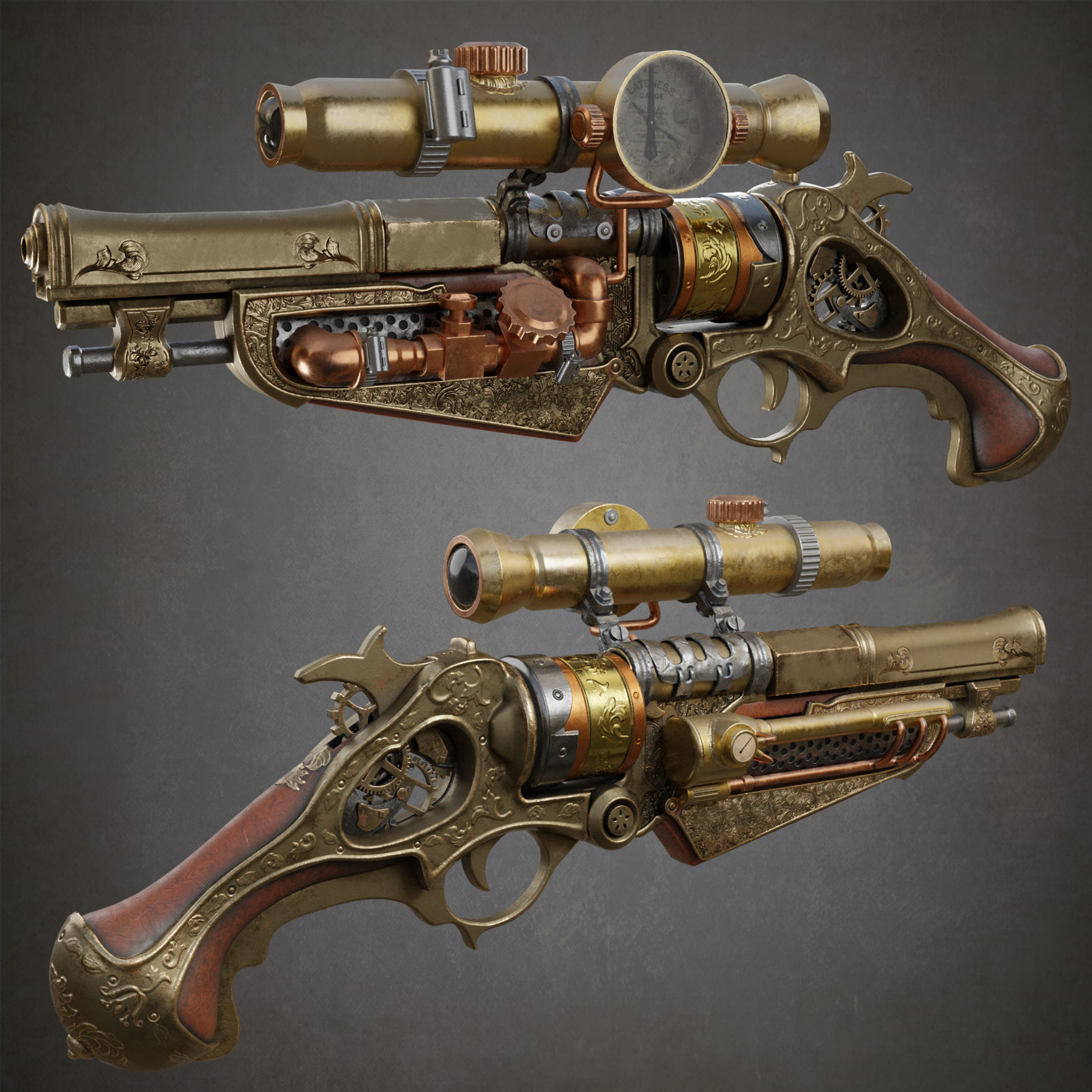This image depicts a steampunk-inspired revolver-style gun intricately detailed with a combination of brass, copper, and gold metalwork. The gun features a large brass scope that spans two-thirds of the length of the top, secured by metal brackets and characterized by bulbous, dark-tinted lenses reminiscent of an old telescope. The scope also includes a compass encased in a silver border. The gun's body showcases a variety of ornamental designs, with elaborate copper piping visible along the side and beneath the barrel.

The short handle is crafted from reddish-brown wood or leather, accented with brass hardware that wraps around it and integrates seamlessly with the trigger and hammer, both of which are also brass. The image, set against a simple dark grey background, displays the weapon from both the left and right side, emphasizing its steampunk aesthetic with additional features like a prominent dial on the side, complete with multiple knobs. The golden and bronze tones of the gun, along with its detailed craftsmanship, give it an antique yet fantastical appearance.